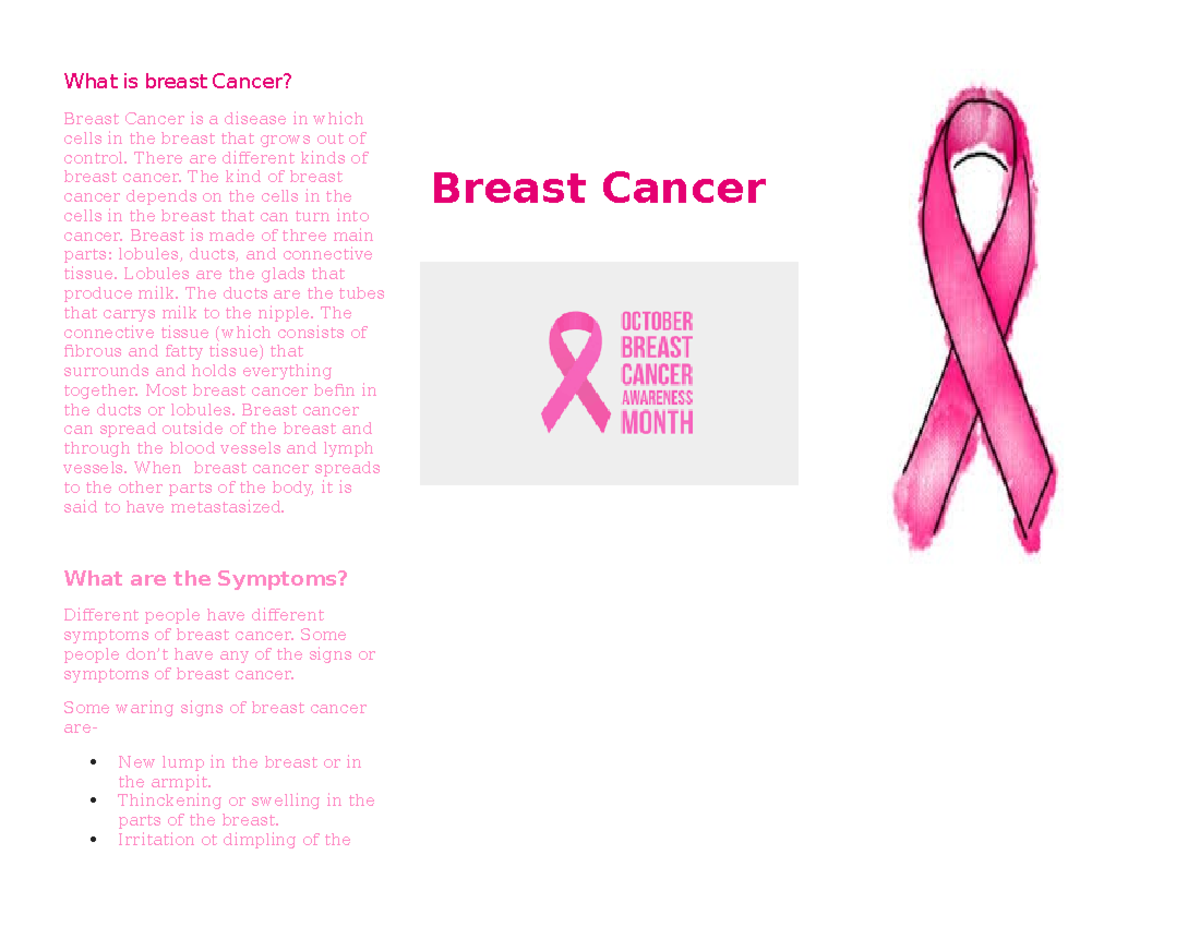The web page has a predominantly pink theme, emphasizing breast cancer awareness. The title prominently reflects "Breast Cancer," accompanied by a smaller graphic that declares "October Breast Cancer Awareness Month." Adjacent to this graphic is a large, striking pink ribbon, universally symbolizing breast cancer awareness.

On the left side of the screen, a comprehensive description of breast cancer is presented. The headline reads, "What is Breast Cancer?" followed by an informative paragraph detailing the condition. The subsequent headline, "What are the Symptoms?" introduces three bulleted symptoms: the emergence of a new lump in the breast, thickening or swelling in parts of the breast, and irritation or dimpling of possibly the breast tissue (the next part of the text is cut off, but it can be inferred).

The entire textual content is in pink font, which, although thematic, may be challenging to read against a white background. The page's two main graphical elements are the folded pink ribbon and a duplicate of the ribbon paired with the "October Breast Cancer Awareness Month" headline. There is no information about the authorship of the page, but it appears legitimate and could be a valuable resource for individuals seeking information about breast cancer.